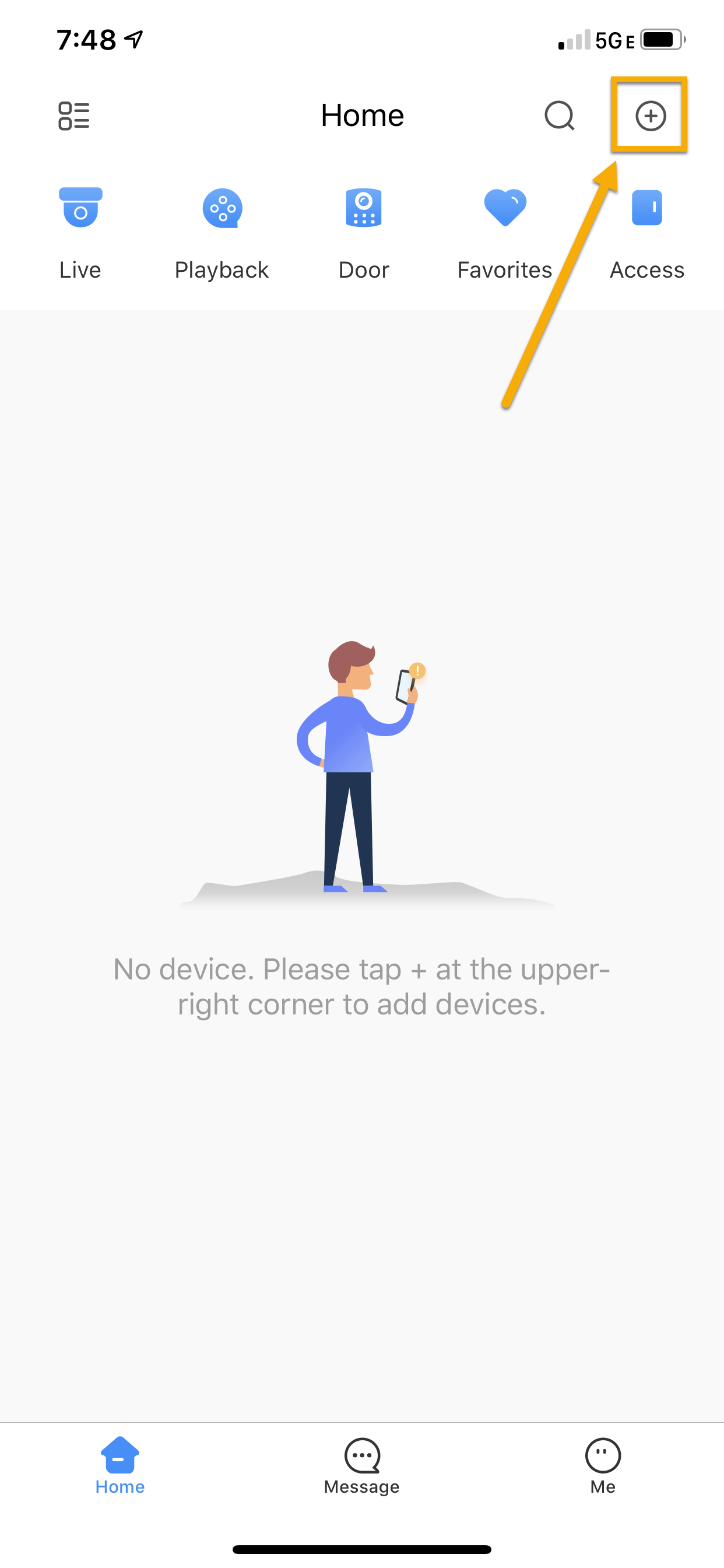A detailed descriptive caption could be:

"The image shows the interface of a home security or Internet of Things (IoT) application. The app utilizes a light theme with a combination of white and light gray tones. The page displayed is titled 'Home,' featuring several icons: 'Live' with a camera icon, 'Playback,' 'Door' with an alarm pad icon, 'Favorites' with a heart icon, and 'Access.' The central section of the screen is empty, displaying a generic cartoon with the message: 'No device. Please tap [+] at the upper right corner to add devices.' This call to action is highlighted with an orange box and an arrow pointing to the plus icon. Along the bottom of the page, there are three tabs: 'Home,' 'Message,' and 'Me,' suggesting the app's functionalities extend across multiple pages, likely relating to home automation and security management."